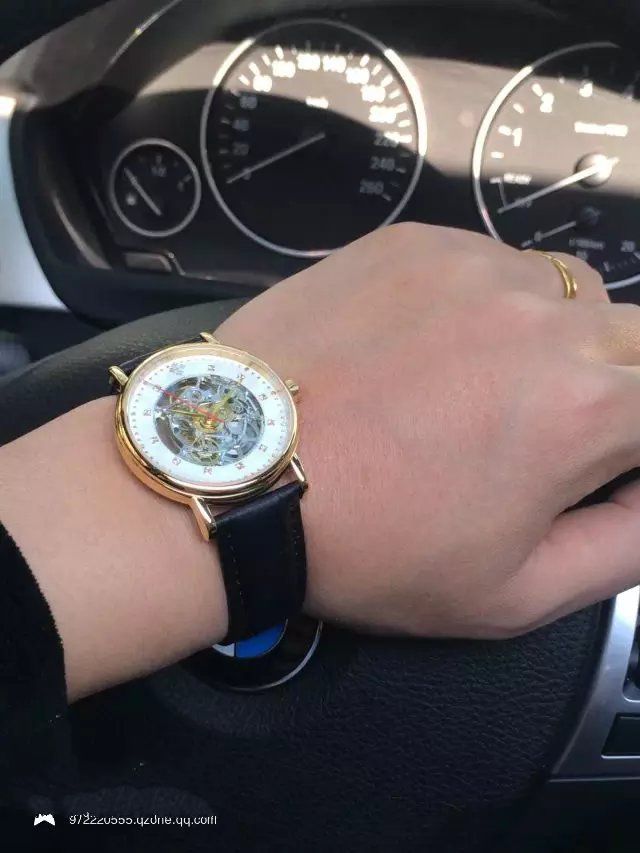The image depicts a man's hand, adorned with a gold wedding ring, resting on the steering wheel of a car. He wears a stylish black watch band with a gold watch, which features a round face. The watch face is predominantly black with a white outer ring and gold-colored numbers. The hand is positioned across the horn area of the steering wheel, prominently displaying a medallion emblazoned with the BMW logo, characterized by its white and blue segments. The car's interior is entirely black with the sun casting its rays directly onto the speedometers, providing a clear view of the instrument panel.